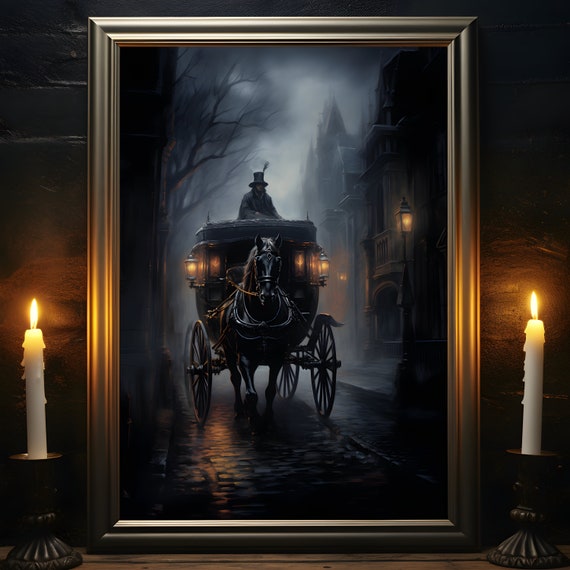This digital photograph captures a beautifully framed painting set against a wall, framed in what appears to be a bronze or gold-colored material—it shimmers due to the candlelight. On either side of the painting are white candlesticks in holders, their flames casting a warm glow. The painting itself is an evocative scene from a bygone era, featuring a black horse-drawn carriage. The carriage, also black, travels towards the viewer along an old-fashioned cobblestone road. Lit lanterns hang on either side of the carriage, emitting a soft orange-yellow light that adds to the painting's nostalgic and atmospheric quality.

The driver, barely more than a shadowy silhouette, wears a top hat and a long black cloak, enhancing the historical ambiance. The backdrop is a foggy night, with faint outlines of buildings along the right side of the road and barren trees on the left, further emphasizing the painting's moody, old-world feel. The damp streets reflect the soft light, adding layers to the misty, nostalgic scene.